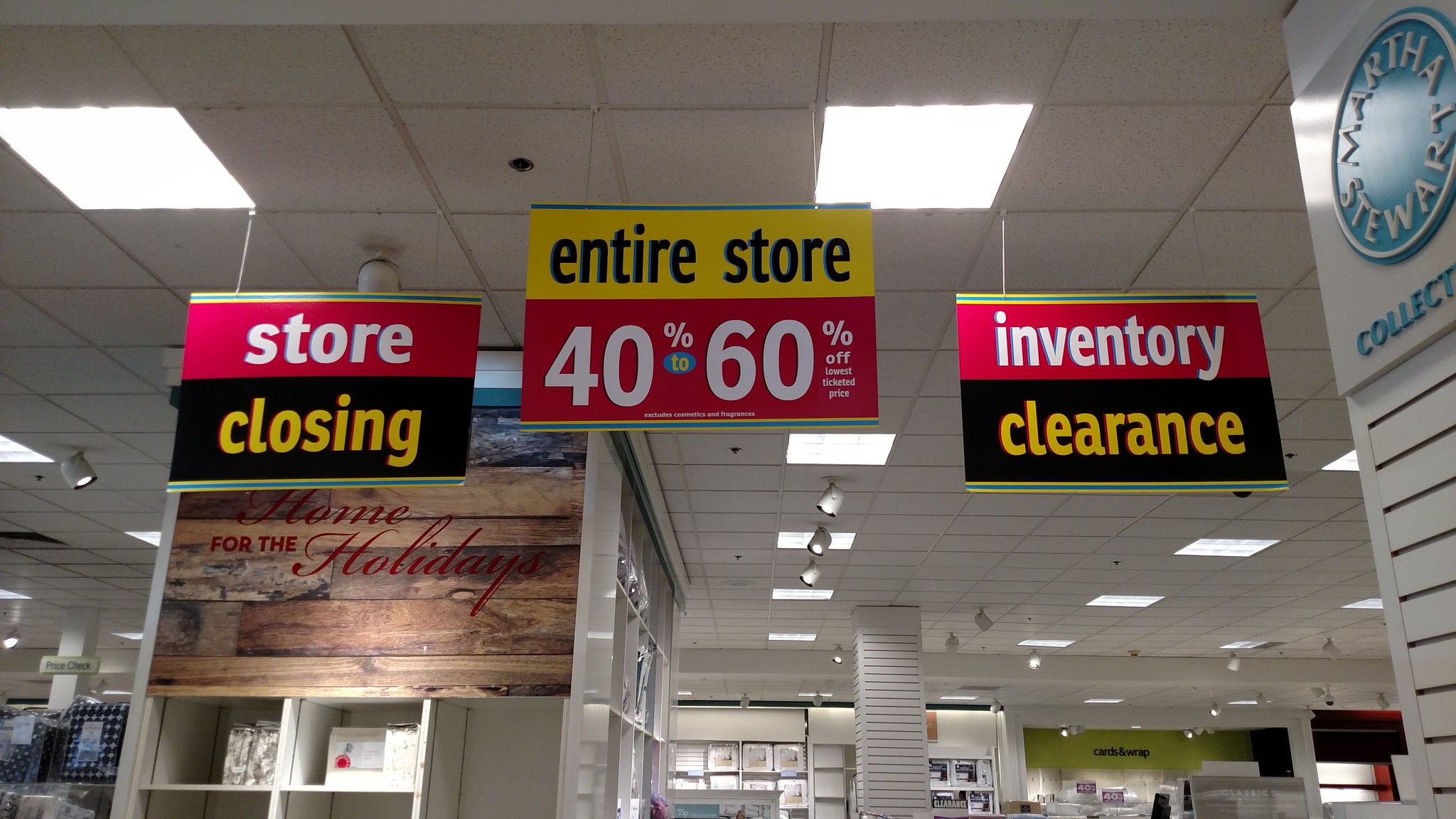This photograph captures the interior of a brightly lit retail store with white tile ceilings and recessed square lights receding into the distance. The main focus centers on three large, rectangular signs hanging from the ceiling, each with vibrant and eye-catching colors. 

To the left, a sign with a black and white background boldly declares, "Store Closing," with "Store" in white font and "Closing" in yellow. The center sign, framed in yellow and red, announces, "Entire Store 40% to 60% Off." The rightmost sign, similarly styled to the left one with a black and red background, reads "Inventory Clearance," with "Inventory" in white and "Clearance" in yellow.

To the right, a circular blue logo features the text "Martha Stewart," partially cut off at the bottom, suggesting it's part of the "Martha Stewart Collection." On the opposite side, an aisle display reads "Home for the Holidays" in red cursive on a slat wood surface, with shelving units below and hard-to-distinguish items, possibly packaged blankets, in the background.

The image overall portrays a bustling store in the midst of a clearance event, highlighted by its organized layout and prominent sale signage.